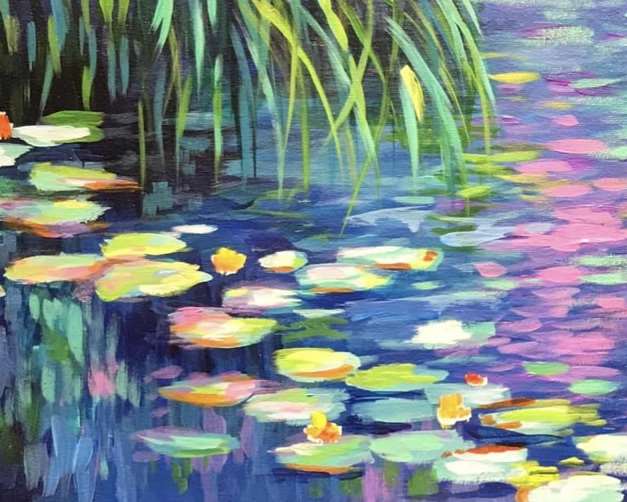This painting depicts an intricate and vibrant pond scene teeming with water lilies. The water, composed of rich blues, greens, and hints of pinks, serves as a canvas for the numerous lily pads floating gracefully on its surface. These lily pads exhibit a spectrum of colors, including light and dark greens, purples, and multicolored combinations with accents of orange, yellow, white, and red. On the top left side of the painting, elongated green and yellow leaves cascade into the water, their vivid hues reflected just beneath the surface. The lilies themselves predominantly appear yellowish-green, with some having delicate yellow and brown flowers, adding to the lush and detailed nature of the scene. Additionally, the reflection of the foliage and lily pads in the pond enhances the painting's depth and realism, capturing the essence of a serene aquatic environment. The artist's technique is characterized by bold, large brush strokes, giving the painting a dynamic and textured feel.